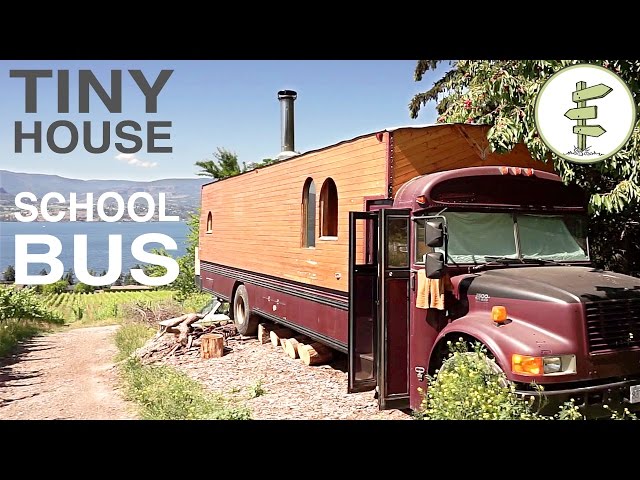In the image to the right, there is a uniquely modified bus that has been transformed into a cozy, tiny house on wheels. The upper portion of the bus features a wooden structure, making it resemble a small cabin perched atop the vehicle. The lower section retains its original design, indicative of either a school bus or a charter bus, distinguished by its burgundy and black color scheme. Atop the wooden cabin-like addition is a black smokestack protruding upwards.

The image is titled "Teeny House School Bus," evident from text in the top left corner. The setting appears to be a serene countryside or camping site, characterized by dirt terrain and extensive green fields surrounding the bus. In the background to the left, a river flows gently through the landscape, adding to the picturesque nature of the scene. Further beyond, majestic mountains rise against a clear, blue sky, completing the idyllic backdrop.